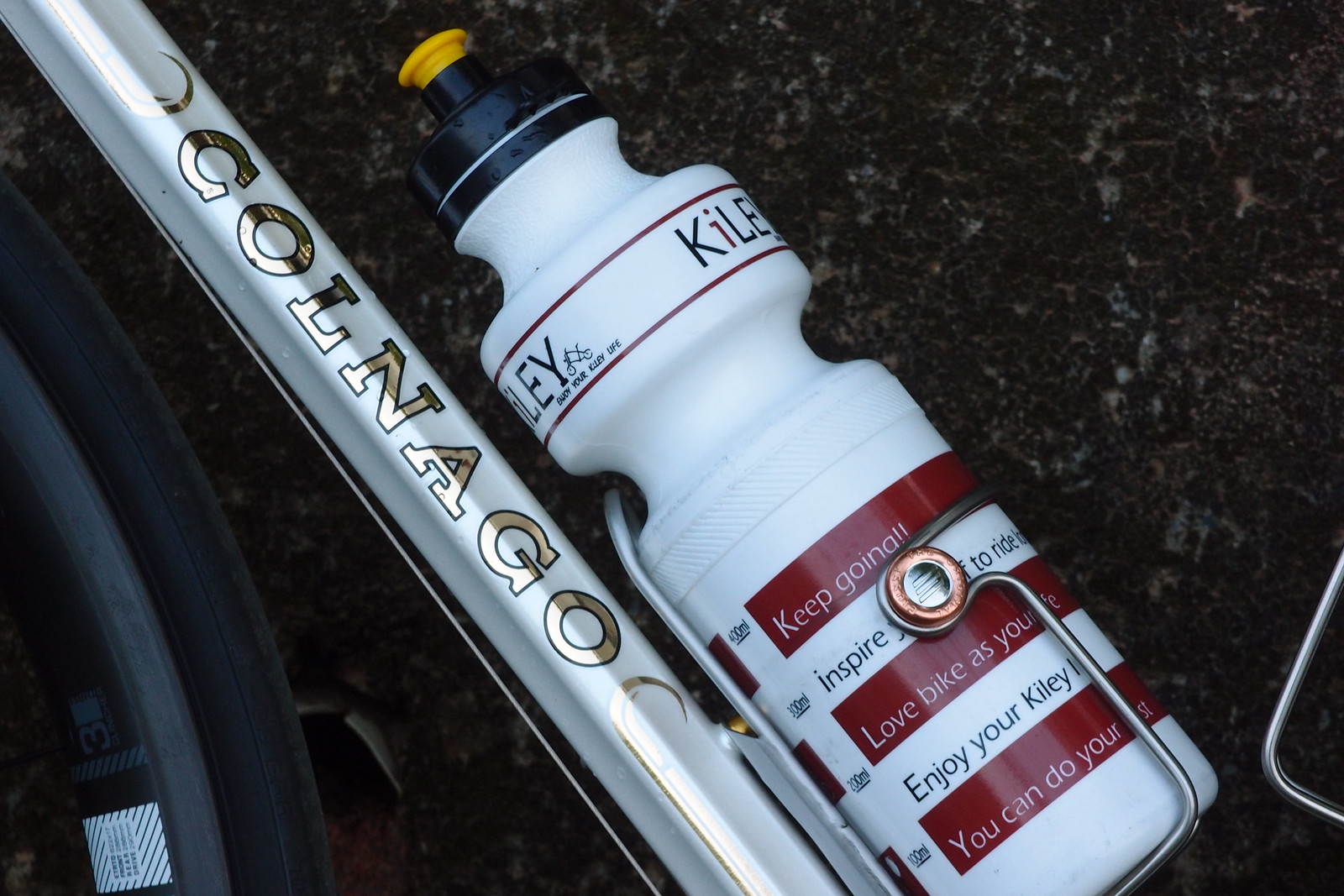In this detailed close-up color photograph, a water bottle is prominently attached to the pearl white frame of a Colnago bicycle, accented by stylish gold lettering spelling out "C-O-L-N-A-G-O." The black tire is partially visible on the left side of the image. The water bottle, mainly white, features a black cap with a yellow pull-top drinking spout. Its base is decorated with alternating red and white stripes, each inscribed with inspirational quotes: "Keep going", "Inspire yourself to ride", "Love bike as your life", "Enjoy your Kiley", and "You can do your best." The photo captures the intricate details and motivational elements designed to encourage the rider.